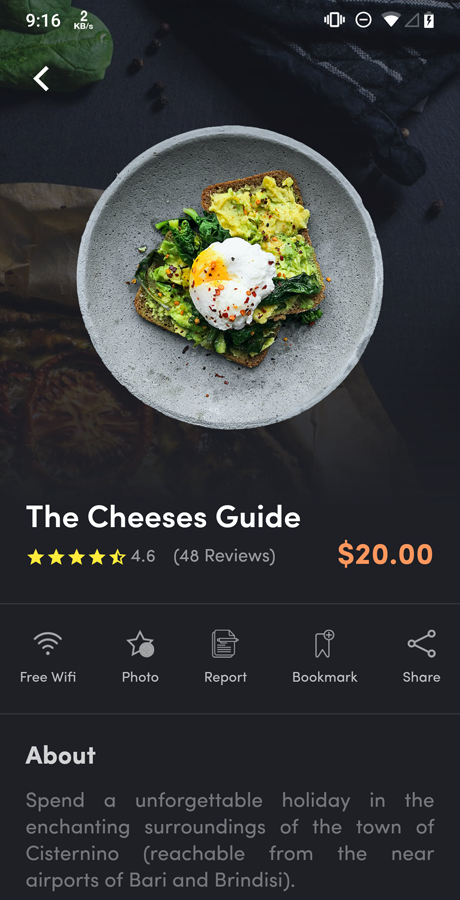Screenshot of a smartphone display showing "The Cheese's Guide" app interface. At the top left corner, the time reads 9:16, while the top right corner displays a fully charged and charging battery icon. 

The main section of the screen features a photograph from a top-down perspective of a gray bowl containing two rectangular slices of brown bread. The bread is spread with a green substance, potentially avocado or kale. Positioned in the center is a white lump with a yellow portion, which appears to be an egg. 

Beneath the photograph, the title "The Cheese's Guide" is prominently displayed, accompanied by a rating of 4.6 stars based on 48 reviews, and the cost listed as $20. 

Below this information, there are five icons with labels from left to right: Free Wi-Fi, Photo, Report, Bookmark, and Share. 

At the bottom of the screen, a brief description reads: "Spend an unforgettable holiday in the enchanting surroundings of the town of Cisternino, reachable from the nearby airports of Bari and Brindisi."